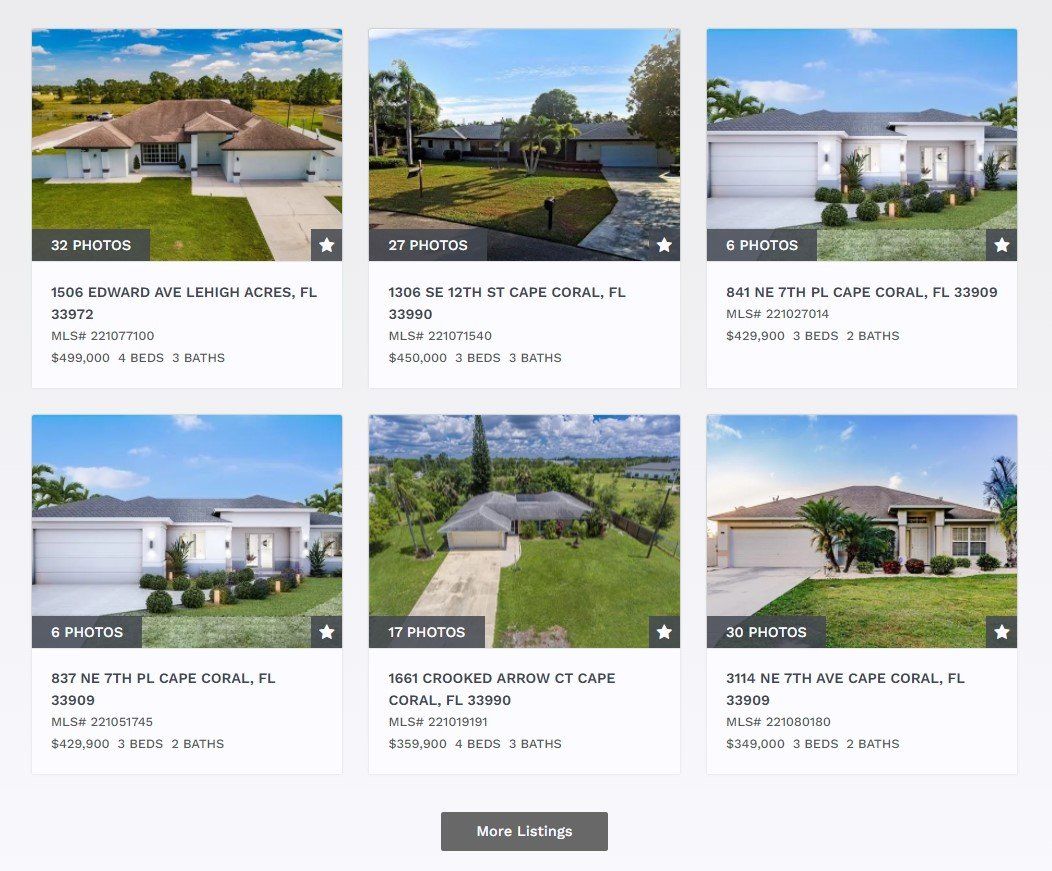A quaint, rustic building standing at the heart of a lush, green meadow, its weathered façade hinting at a rich history. The structure, subtly integrated into its natural surroundings, is enveloped by vibrant grass that stretches out in every direction, painting a serene and picturesque landscape.